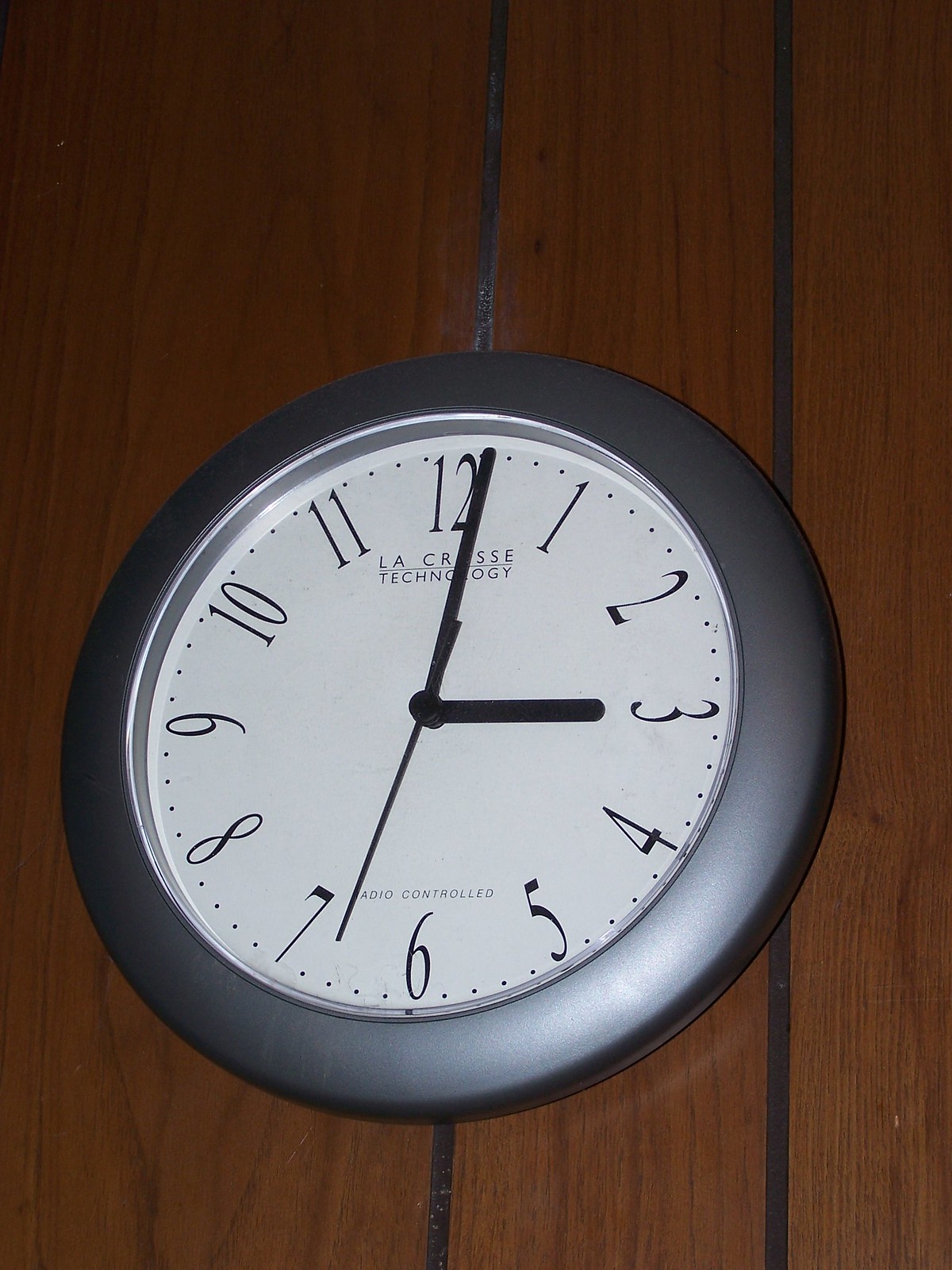The image shows a La Crosse Technology radio-controlled clock mounted on a wall with dark paneling reminiscent of 1970s interior design. The clock is illuminated from below, casting a subtle glow upwards and highlighting its features. The clock's frame, designed to mimic chrome but likely made of dull gray plastic, surrounds a white face with a modern font. All twelve numbers are displayed clearly and remain upright around the circular display. The clock features black hour, minute, and second hands, contrasting sharply against the white background. Minute markers are indicated by small dots around the perimeter, adding to its contemporary look.